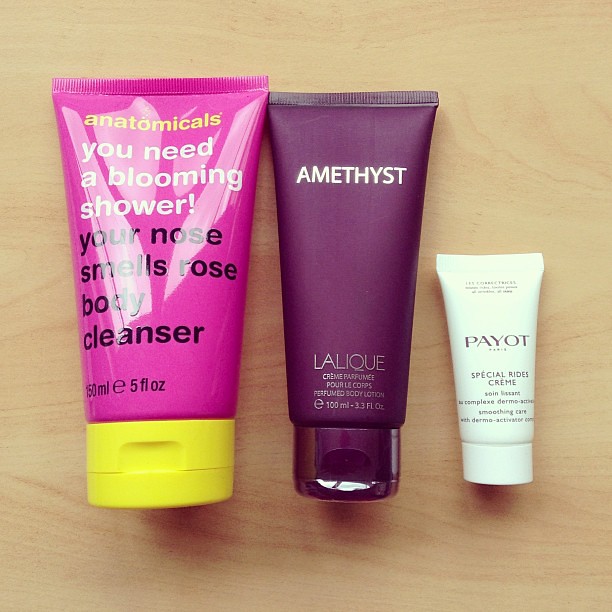The image showcases three cosmetic tubes neatly arranged on a light brown wooden surface. The largest tube, positioned on the left, is a vibrant hot pink with a contrasting yellow cap. It features the brand name "anatomicals" in yellow, followed by the product name "You need a blooming shower" in white letters, and the description "Your nose smells rose body cleanser" in black, with a volume of 50 milliliters (5 fluid ounces). The central tube boasts a rich purplish-maroon color with "amethyst" written in silver, and below that, the brand name "Lalique" along with the description "cream perfume. Pour le corps, perfume body lotion," in smaller print, indicating a volume of 100 milliliters. The smallest tube on the right, which is white, bears the brand "Payotte" in grayish-purplish letters, alongside the product name "special rides cream," further described as "smoothing care with dermal activator." All three beauty products are meticulously displayed for easy viewing and comparison.